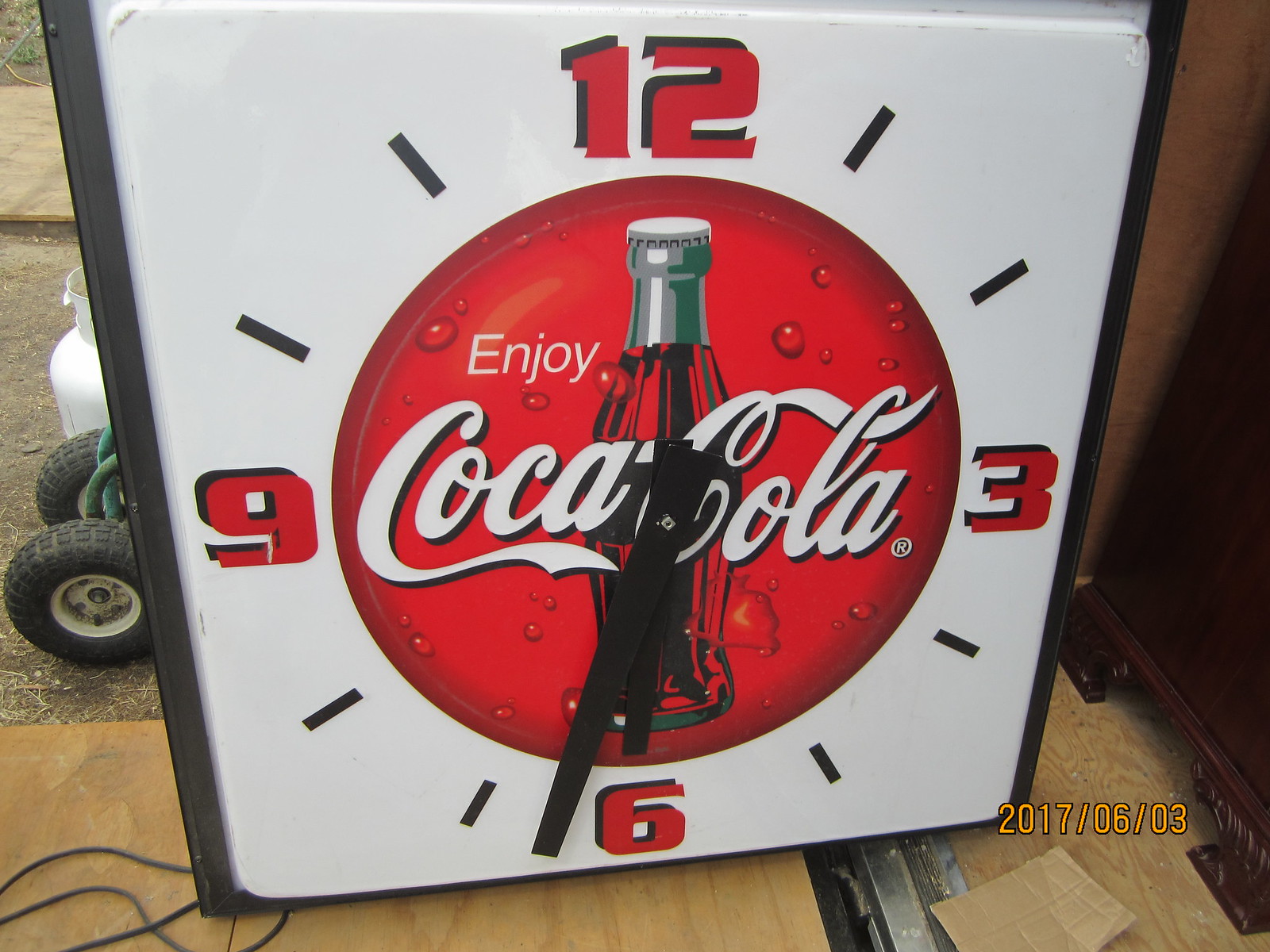In the foreground, a set of black rubber wheels are visible, likely attached to some kind of mobile object or equipment. Beside the wheels, there is a white propane tank placed on a dirt ground. The scene also includes a wooden countertop, where a vintage Coca-Cola clock is prominently displayed. The clock, with a red background, has the words "Enjoy Coca-Cola" inscribed at its center, which also features a miniature glass Coca-Cola bottle with a silver top. The clock's face shows the numbers 12, 3, 6, and 9, with two dash marks between each numeral for the remaining hours. The clock’s minute hand is pointed at the positions 1, 2, and 6, while the hour hand points towards 1, 8, and 6, drawing attention to the nostalgic theme centered around Coca-Cola memorabilia.